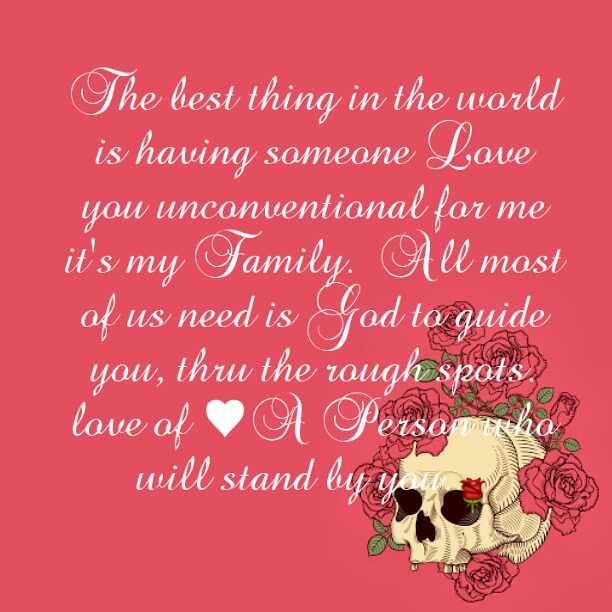The image is set against a hot pink background and features a cursive white text quote, though the quote's structure is somewhat jumbled. It reads, "The best thing in the world is having someone love you unconditionally. For me, it's family. All most of us need is God to guide you through the rough spots. Love of ♥, a person who will stand by you." 

The text appears degraded and low-quality, possibly due to being over-sharpened and copied multiple times. The bottom right corner contains an intricate piece of artwork: a cream-colored skull adorned with hot pink roses and green leaves, which extend from all sides of the skull. The vivid colors of the roses complement the hot pink background, adding a striking visual element to the overall design.